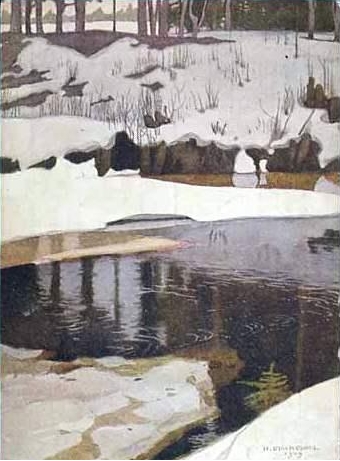This is a vertical painting depicting a serene, snowy winter landscape dominated by shades of white, brown, tan, and muted gray tones. The foreground features a dark brown pond that appears strikingly realistic, with visible ripples and reflections of thin tree trunks sprouting up from the surrounding terrain. The water, partially frozen over, also reveals bits of vegetation underneath its surface.

Patches of snow cover the ground in the front, while dense, pure white snow blankets the middle section, creating a visually stark contrast against the brown landscape. The scene also includes dried grasses peeking through the snow, adding texture and depth. The backdrop transitions from the snowy hills into a forest where the thin trunks of trees, possibly birch, reach upward.

In the distant background, faint, hazy mountains can be seen peeking through the gaps between the trees, adding a sense of depth and expanse to the composition. The overall atmosphere of the painting is tranquil and muted, effectively capturing the calm and stillness of a snowy winter day.